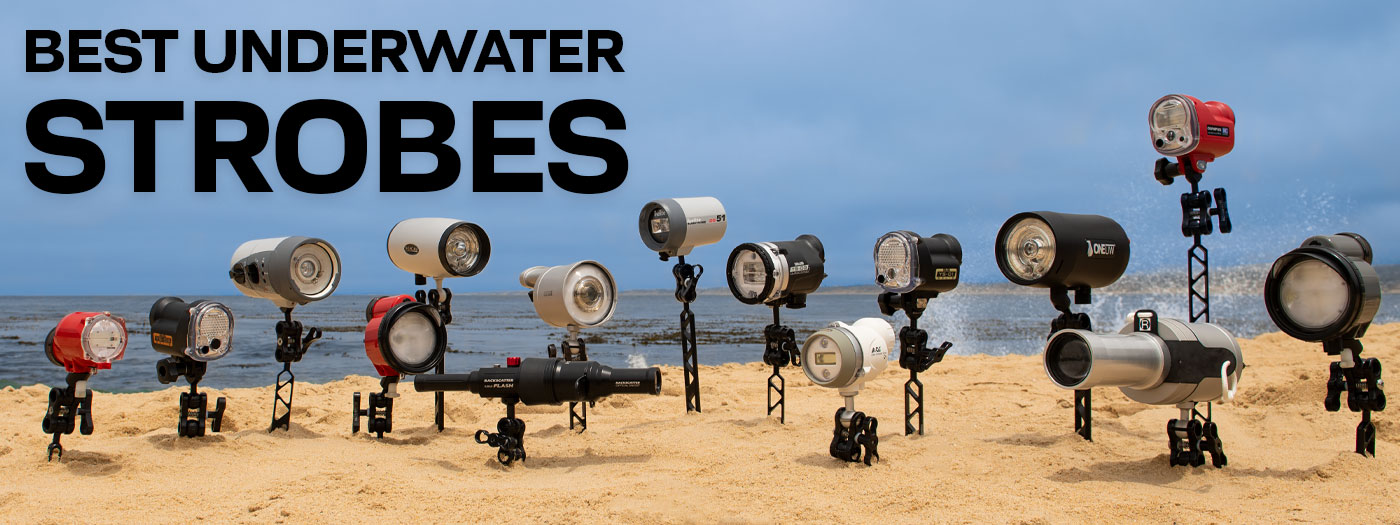This panoramic image showcases a collection of 15 underwater strobe lights arranged in the sand on a beach. The strobe lights come in various colors including red, white, silver, and black, and display different sizes and shapes of lenses, some of which are elongated. Above the scene, the caption "Best Underwater Strobes" is prominently featured in the top-left corner, with the word "strobes" standing out in larger text. In the background, the vast ocean extends towards the horizon, meeting a clear, open sky. The strobe lights are not connected to any visible power source, adding a mysterious element to their orderly arrangement on the beach.